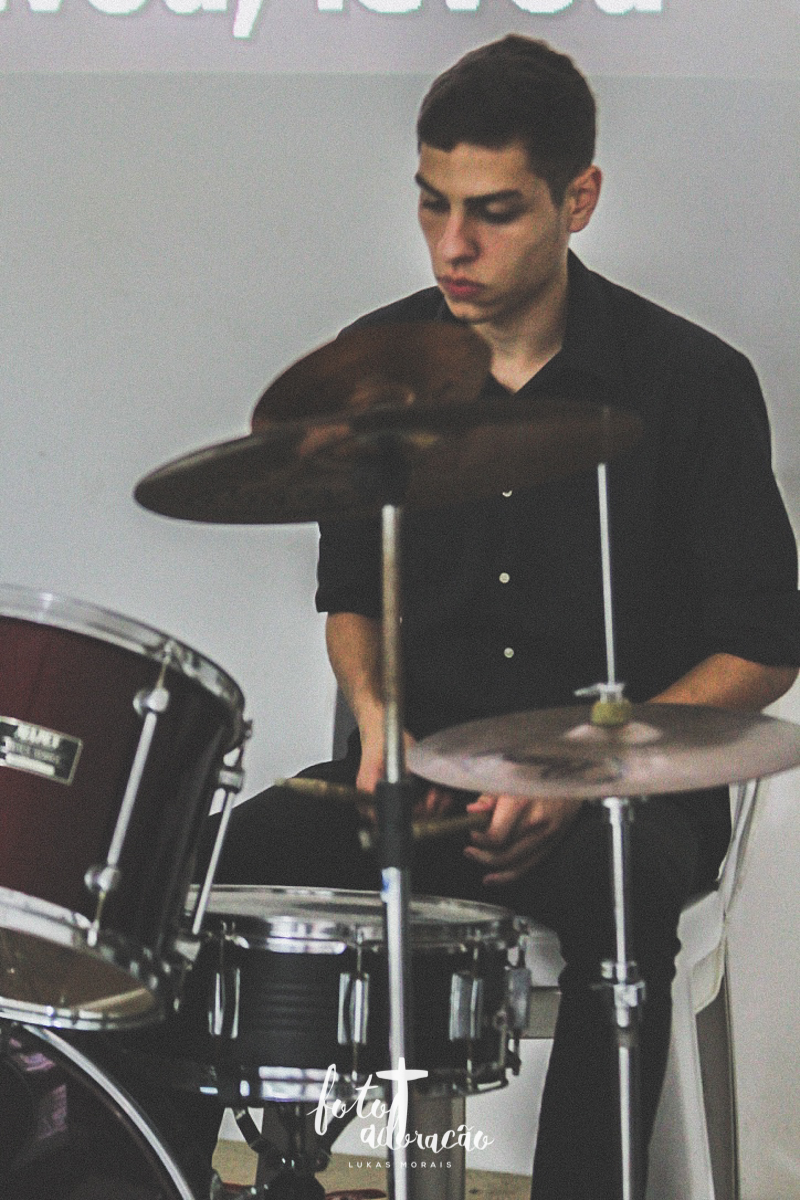The photograph captures a young male drummer, likely in his late teens or early twenties, deeply engrossed in his performance. He has short brown hair and sharp features, and he is wearing a black button-up shirt with the sleeves rolled up to the elbow paired with black pants. Seated on a white chair against a white backdrop, his eyes are focused downwards at the drum set located towards the bottom left of the image. Both of his hands hold light brown drumsticks, which are striking a snare drum. The drum set, composed of a mix of black and dark red drums, features bronze-colored cymbals mounted on silver stands that somewhat obscure his body. The text "FOTOADORACAO" is imposed in white at the bottom of the image, suggesting it could be a watermark or part of an advertisement.